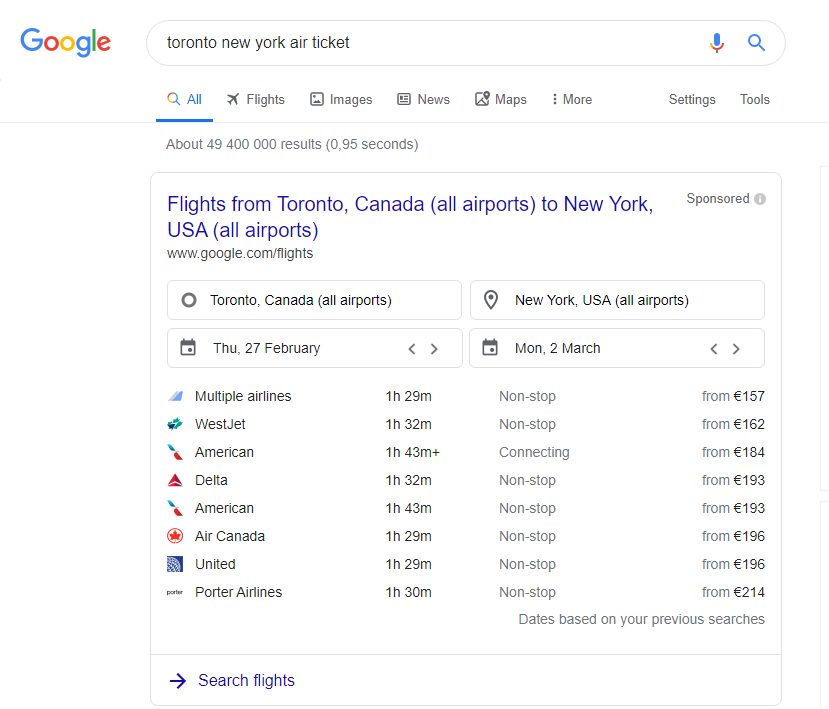The image displays a Google search results page for the query "Toronto, New York air ticket." The search bar at the top of the page contains this query, and beneath it are tabs labeled "All," "Flights," "Images," "News," "Maps," "More," "Settings," and "Tools." The search results show that there are approximately 49,400,000 results and the search took about 0.95 seconds. 

The highlighted section in the results provides specific flight options for a trip from Toronto, Canada (all airports) to New York, USA (all airports) with travel dates listed as Thursday, February 27th to Monday, March 2nd. 

The detailed flight information includes:
- Multiple Airlines: 1 hour 29 minutes, non-stop, starting from 157 Euros.
- WestJet: 1 hour 32 minutes, non-stop, starting from 162 Euros.
- American Airlines: 1 hour 43 minutes, connecting, starting from 154 Euros.
- Delta Airlines: 1 hour 32 minutes, non-stop, starting from 193 Euros.

All the information is sourced from Google at www.google.com.